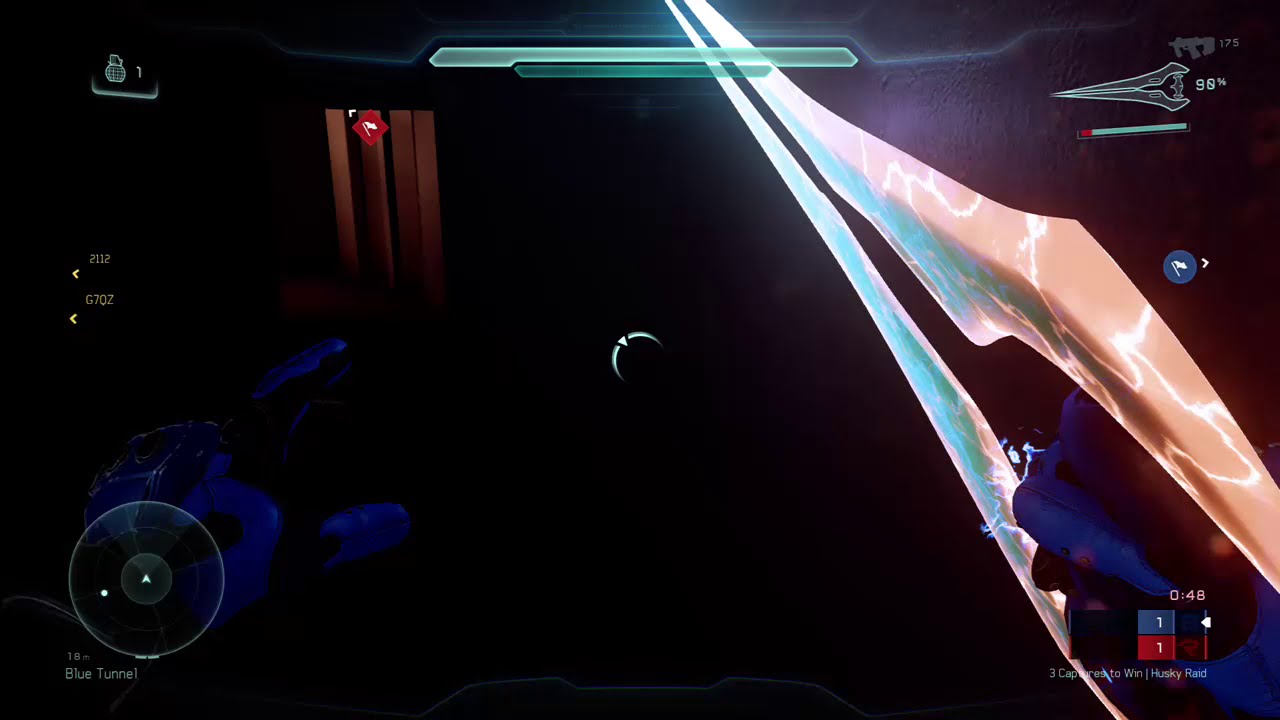This image is a detailed video game screenshot, potentially from the game Halo. The scene appears to be viewed from the first-person perspective of a character wielding a futuristic sword. The right side of the image is dominated by a hand holding a sword that extends out to a point, with hollow spaces in its blade, appearing like two parallel lines converging into sharp tips. The hand is covered in a bright blue glove with black trim.

In the top right corner, there is an icon of a sword, likely indicating the weapon being used, and below it, there is a display showing the weapon's strength as a percentage. The upper left corner features an icon for a grenade and a health bar, maintaining the player's status information.

The bottom of the image provides additional information: the bottom left corner displays a radar-like circle, perhaps indicating a map, while the bottom right corner includes various text and numbers, such as "1, 2, 1, 1, 2, G, 7, Q, Z, 48," likely representing gameplay mechanics or scores. Specifically, the number 48 stands out prominently here.

The image predominantly uses dark colors, with a palette that includes black, red, blue, brown, green, salmon, and light purple. Light streaks, resembling lightning bolts, add dynamic elements to the scene, and a beige-pink lightning bolt with white streaks further enhances the dramatic effect. The background is largely indistinct due to darkness but features hints of a shiny light purple wall on the right. The environment is likely indoors, characterized by hanging plastic flaps on the left, suggesting a doorway.

Overall, the scene's emphasis is on the action and HUD (Heads-Up Display) elements typical of a combat video game setting.